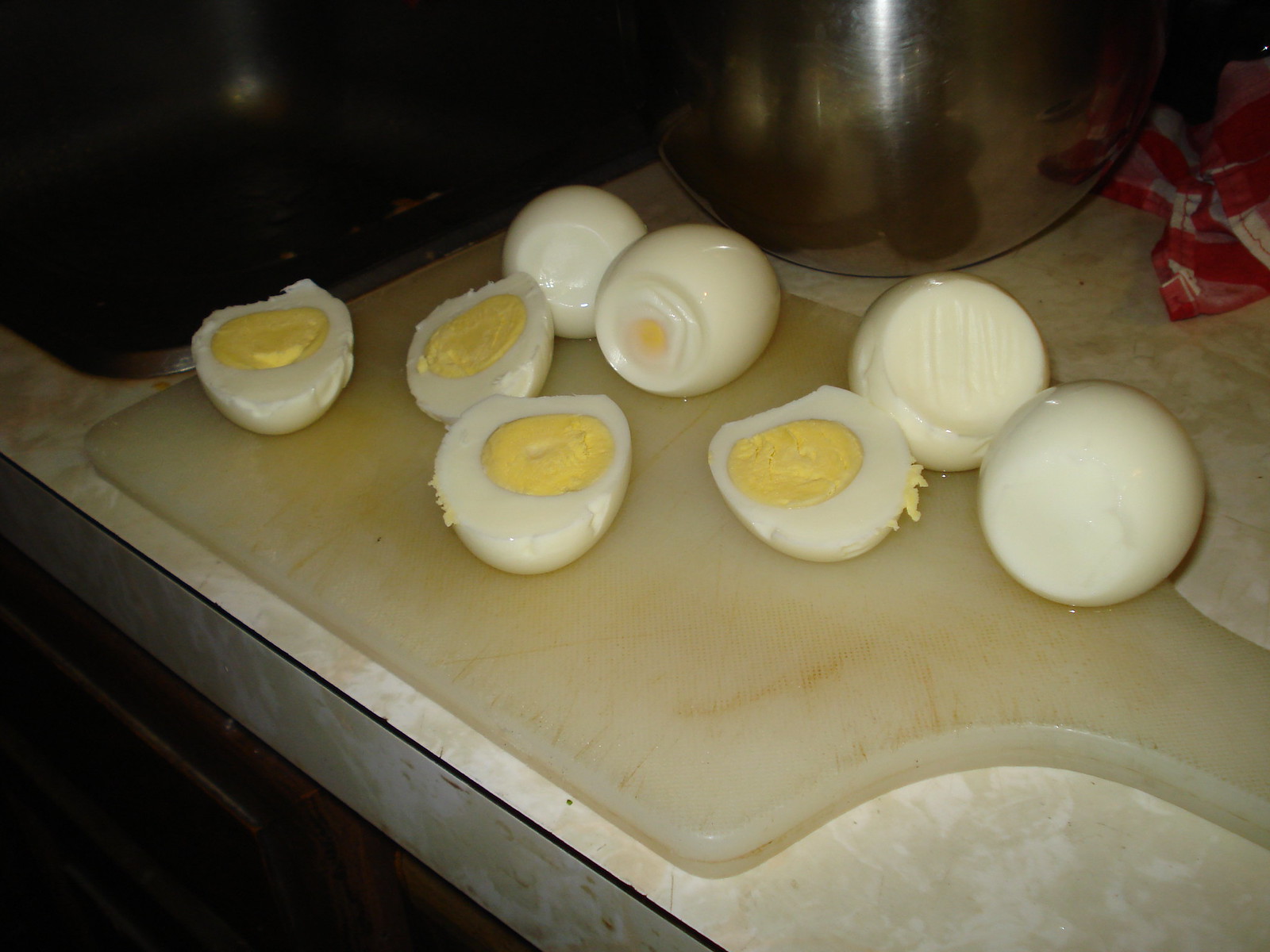The photograph depicts a busy kitchen scene with a worn, white plastic cutting board placed on a Formica marble-look countertop. Resting on the cutting board are four whole hard-boiled eggs, along with two hard-boiled eggs that have been cut in half, revealing their yolks. The cutting board appears weathered and stained from frequent use, with some liquid still present, indicating the eggs were recently boiled. To the right of the cutting board is a stainless steel bowl, possibly used during the egg preparation. The background features brown cabinets and a blurred view of a stovetop, highlighting an active kitchen environment.